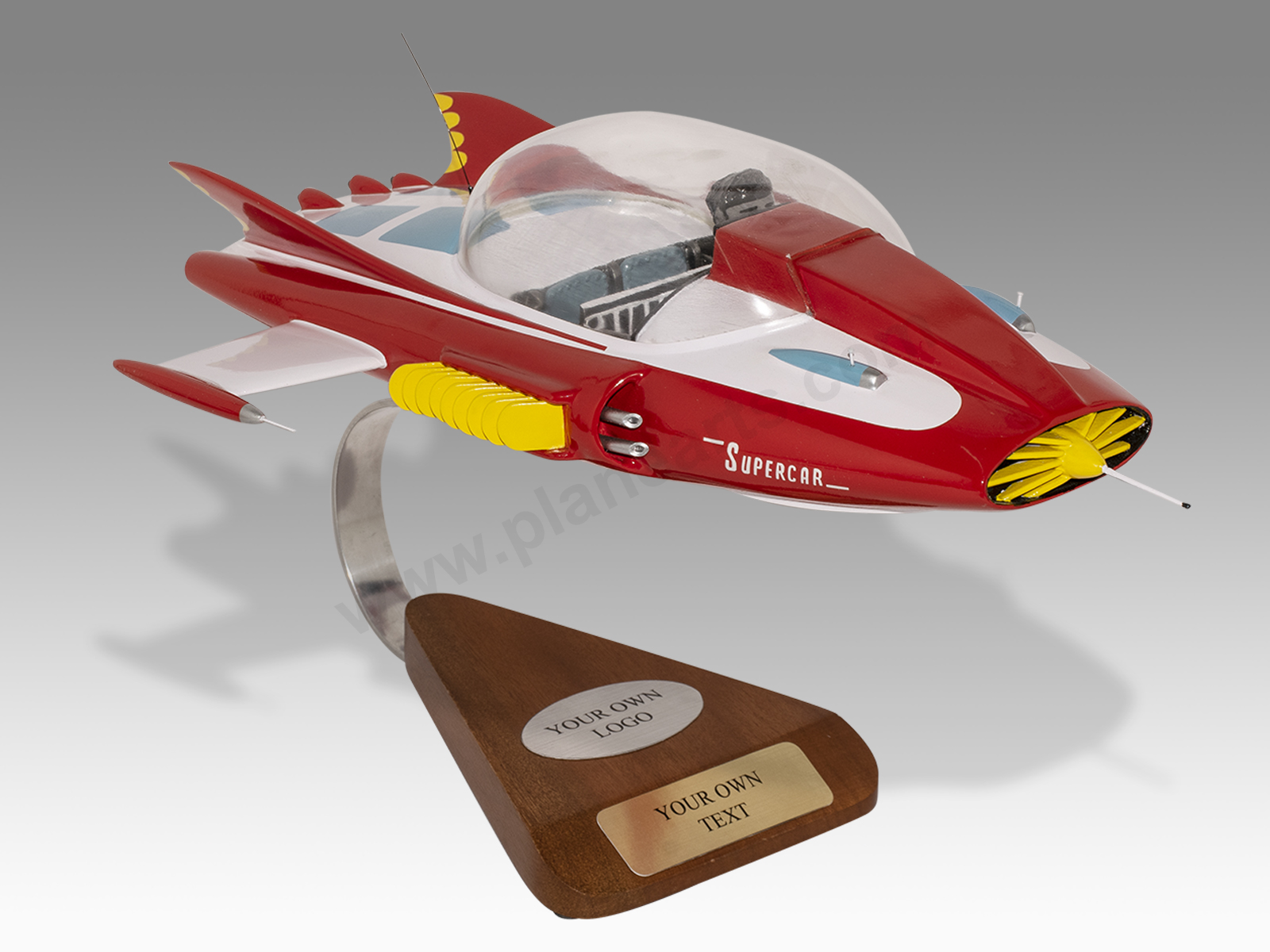The image showcases a detailed model of a customizable futuristic spaceship-car hybrid, prominently displayed against a plain white and gray background, suggesting a product photograph. The spaceship, primarily red with yellow, white, and blue accents, features a clear cockpit dome reminiscent of a retro-futuristic vehicle design. It includes a front yellow propeller with an antenna, side yellow details, red-edged wings with pointed tips, and a rear spoiler trimmed in yellow. The body of the spaceship bears the word "supercar" in white font on its side.

The model is mounted on a triangular wooden stand, bolstered by a silver metal stem. Attached to the stand are two customizable plaques: the top plaque, circular and silver, reads "your own logo," while the forward-facing golden plaque reads "your own text." There is also a faint watermark in the background, partially obscured but hinting at a planet-themed logo or website. The overall presentation, including shadows cast by the spaceship, suggests this product is intended for a business to personalize, possibly as a unique award or desk ornament.